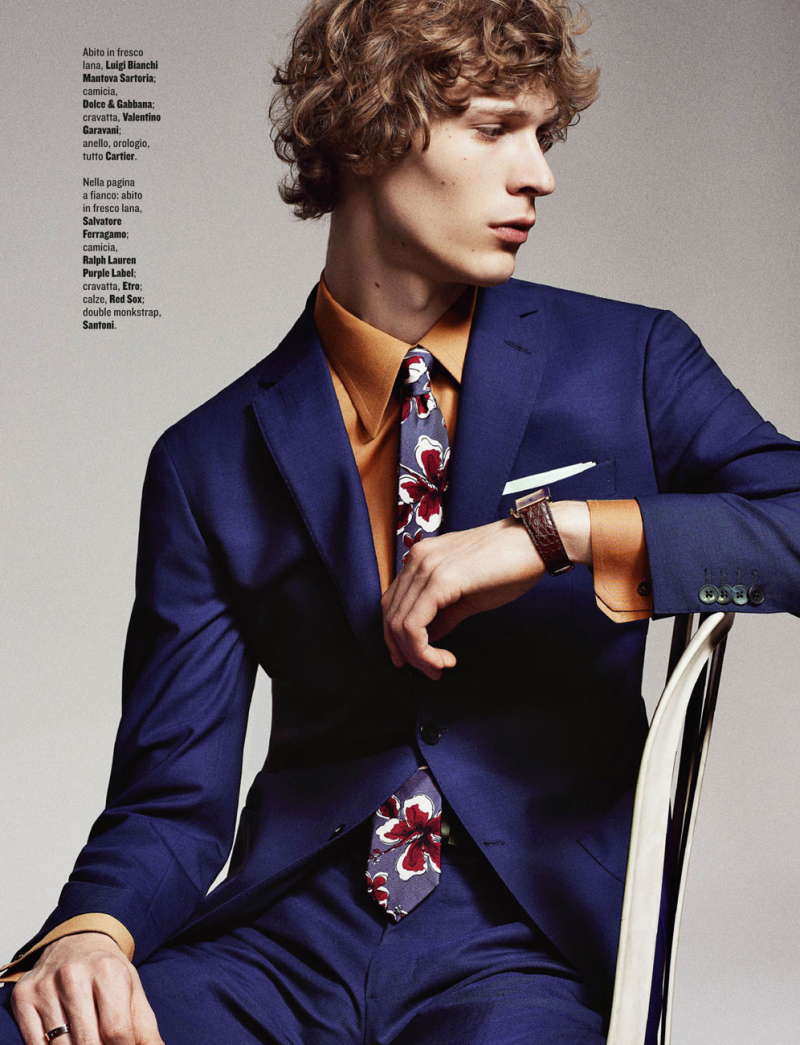The image captures a young Caucasian man, approximately 18 years old, with a slim build and high cheekbones. He has curly medium-length brown hair that reaches about to his jawline. He is sitting sideways on a white chair with a black frame, his body facing the camera but his head turned to look to the right side of the image. He is wearing an elegantly tailored dark blue suit with matching trousers, a muted orange dress shirt, and a floral tie featuring bright red and white flowers on a light blue background, possibly hibiscus.

His right hand, which sports a single band ring, rests on his right knee while his left arm is angled at 45 degrees, resting on the backrest of the chair like an armrest, showcasing a brown leather wristwatch. The background is a solid gray, creating a sleek and minimalist backdrop.

In the upper left corner, there is small, black text listing various designer brands, but it is too small to be legibly read. Despite this, the brands mentioned include Blanchi, Ceteria, Dolce & Gabbana, Valentino, and others. The young man is distinctly positioned to emphasize not only his attire but also the accessories, particularly the watch, suggesting a modeling or fashion-oriented photoshoot.